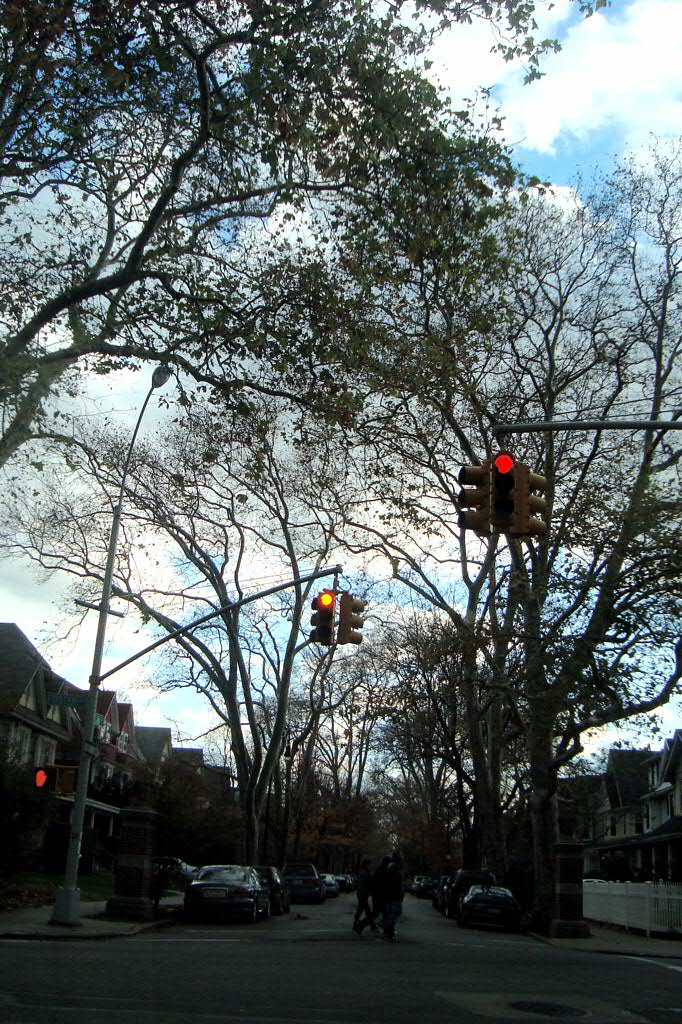The photograph captures a residential neighborhood street scene. Lined with houses and apartments on both sides, the street has numerous cars parked along the curb. Dominating the foreground, two traffic lights both display red, signaling vehicles to stop, while a red hand on a walking sign to the left flashes "don't walk." The perspective of the image is from a ground view, looking slightly upward. This angle prominently features a bright blue sky filled with white, fluffy clouds and interspersed with the branches and leaves of numerous trees. Mid-picture, there's a faint, possibly overexposed figure that might be on a motorcycle or a bicycle, waiting at the light. A white picket fence runs along the right side of the street. Additionally, four figures, possibly kids or adults, can be observed in the midst of crossing the street.